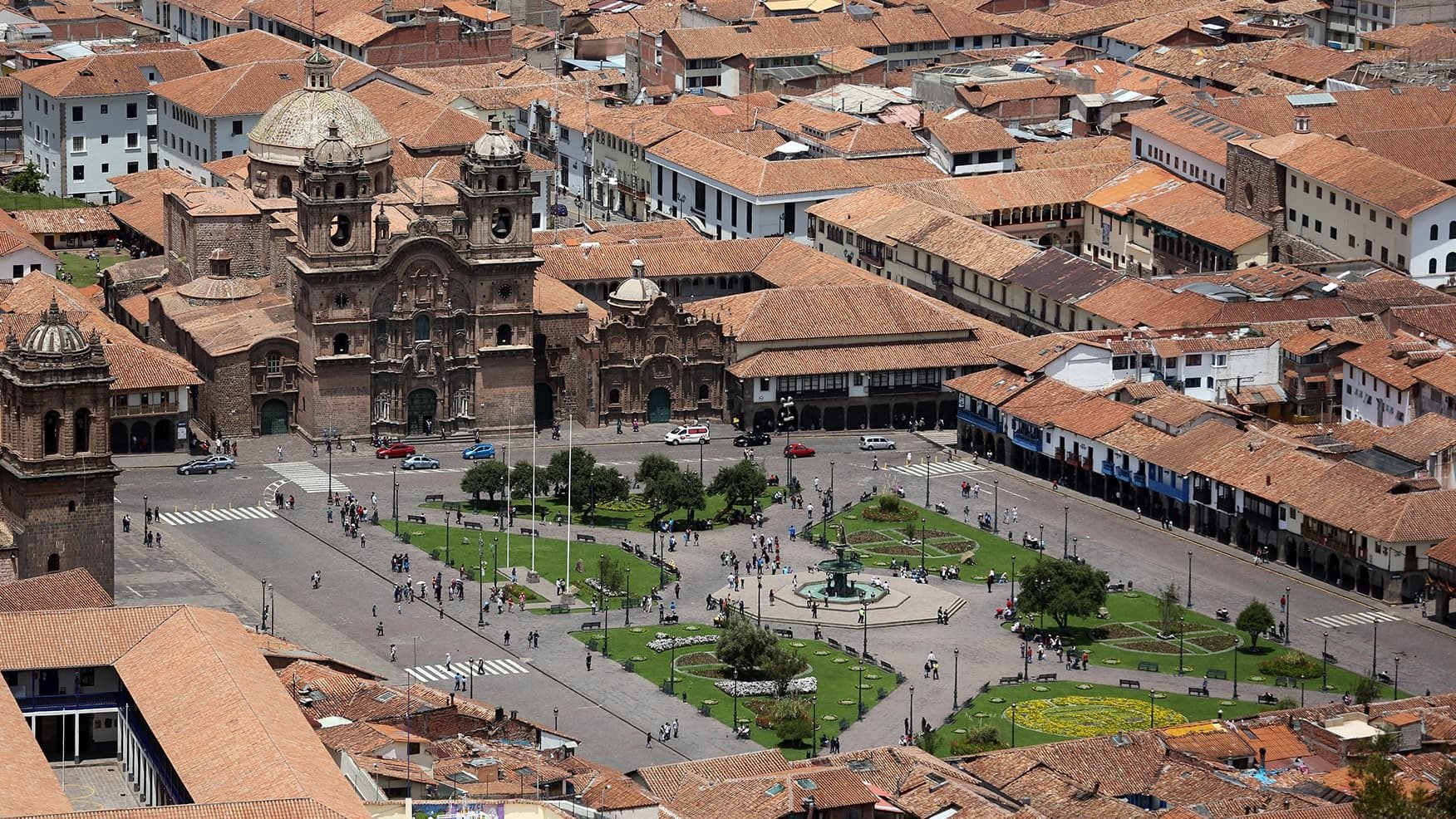The image, captured from a high vantage point such as a drone, showcases a bustling town center during the daytime. The scene is dominated by a prominent building with a distinctive dome and ornate front, resembling a grand cathedral or an important government structure, positioned towards the top of the central square. Surrounding this grand edifice are numerous houses with brown roofs, densely packed along the street. The wide horizontal rectangular frame reveals a spacious plaza or park in the middle of the town, featuring a dark gray pavement and patches of green grass. In the heart of this open space lies a picturesque fountain with a teal pool and an intricate statue emitting water. People can be seen strolling along the pathways and sitting on benches, contributing to the lively atmosphere. Streets extending from the sides of the square host cars and pedestrians, integrating the serene park setting with the dynamic daily life of the town.